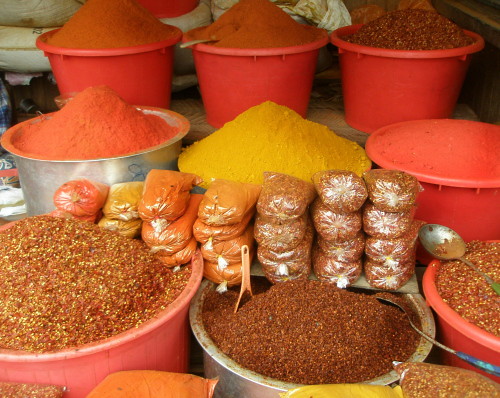In this vibrant street market scene reminiscent of Indian spice shops, a tiered shelving unit displays a tantalizing array of spices in large bins and buckets. There are nine prominent bins, most of which are plastic, with at least two being metal. Each bucket is heaped to the brim with colorful spices including shades of brown, orange, yellow, and a striking deep pink. One central bin, containing a bright yellow powder that resembles turmeric, stands out against the backdrop. Nestled between these bins are pre-packaged bags of the spices, neatly arranged for sale. The overall tableau is bustling with vivid hues and the rich textures of the spices, promising an aromatic allure. In the upper left corner, a white PVC pipe subtly peeks into the frame, adding an incongruous but interesting touch to this exotic market display.